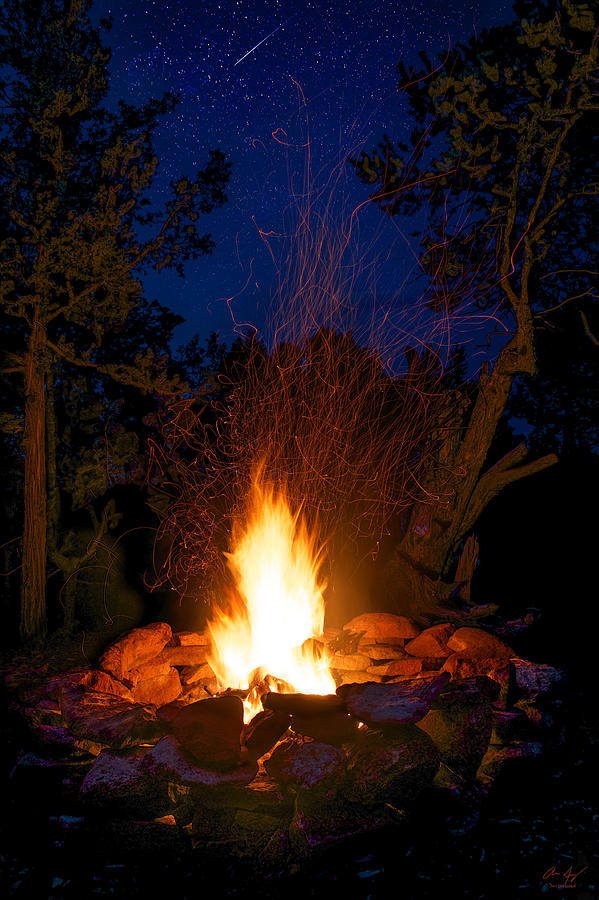Against the backdrop of a dark blue night sky filled with stars, this photograph captures a blazing campfire surrounded by a circle of stacked rocks. The fire's bright orange flames reach high into the air, creating a dynamic visual focal point. The image appears to be a time-lapse, as sparks from the fire form intricate, fiery red trails, adding a mesmerizing effect reminiscent of squiggling lines or a delicate drawing etched into the night. Evergreens frame the scene, their foliage partly illuminated by the fire, casting a green hue against the dark. Among the stars, a streak of white suggests a comet or falling star, enhancing the ethereal quality of the night. The photograph's vertical orientation contributes to the impression of height in the flames and the vastness of the night sky, making it detailed, vivid, and captivating.